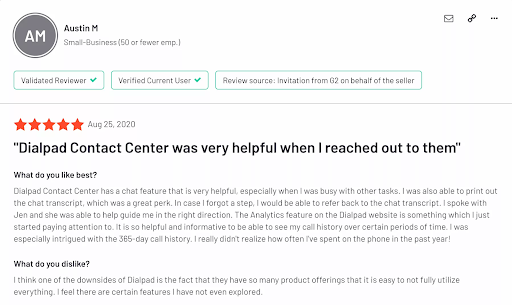Here is a detailed, cleaned-up caption for the review image:

---

The review features a minimalistic white background with black and dark gray text. In the upper left-hand corner, there is a gray circle outlined by a gray line, containing the white capital letters "A" and "M" at its center. Adjacent to this circle is the reviewer’s name, "Austin M," followed by the text "Small Business, 50 or fewer employees." Directly below this information, there are three green-outlined rectangles with green check marks, each indicating specific credentials. The first rectangle says "Validated Reviewer," the second reads "Verified Current User," and the third states "Review Source: Invitation from G2 on Behalf of the Seller." Beneath these details, a thin gray line separates the credentials from the review content.

The review prominently features five red stars, indicating a high rating, followed by the date "August 25, 2020." In bold text and enclosed in quotation marks, the review begins with: “Dialpad Contact Center was very helpful when I reached out to them.” Following this, the section titled "What do you like best?" presents a detailed paragraph of text highlighting the user's positive experiences. Further down, the section "What do you dislike?" contains two sentences that discuss any negative aspects encountered by the reviewer.

---

This revised caption provides a comprehensive and structured description of the review image, covering all its key elements in a clear and detailed manner.